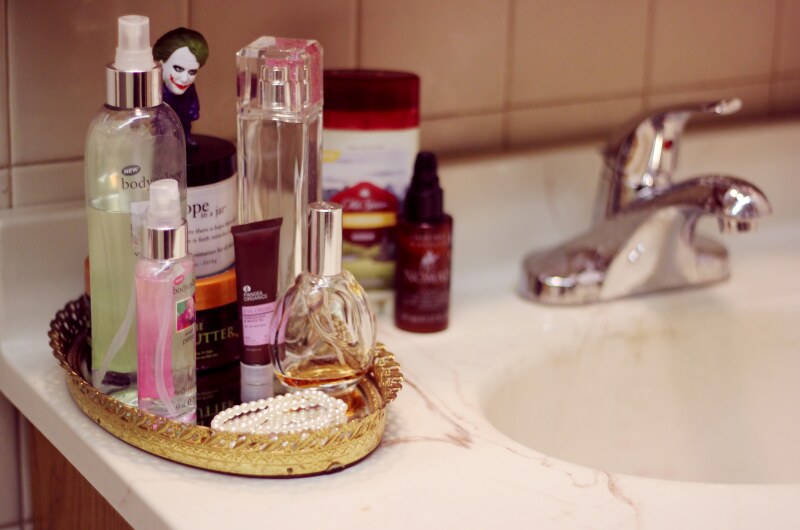In this close-up, landscape-oriented photograph, the focal point is a sophisticated marble sink showcasing prominent brownish streaks amidst its white base. The sleek, silver faucet, crafted from stainless steel, features a top-mounted handle that lifts to adjust water pressure and turns left or right for hot or cold water selection. Integrated seamlessly into the countertop, the bowl of the sink mirrors its marble material.

A white tile wall forms the backdrop, while the countertop itself is wooden, adding a rustic charm to the setting. On the left side of the sink, a gold-toned basket – possibly metal or wood – holds a variety of toiletries. Among these is a tall, clear bottle with a yellow liquid labeled "body" (the remainder obscured), a clear spray bottle with pink accents and transparent liquid, a string of pearls, an almost-empty circular glass perfume bottle containing brown liquid, and a tall, skinny, clear rectangular bottle showing no visible liquid content. A brown lotion bottle and a container of Old Spice complete the ensemble. This meticulous assortment of items, paired with the elegant sink design, captures a blend of luxury and practical utility.